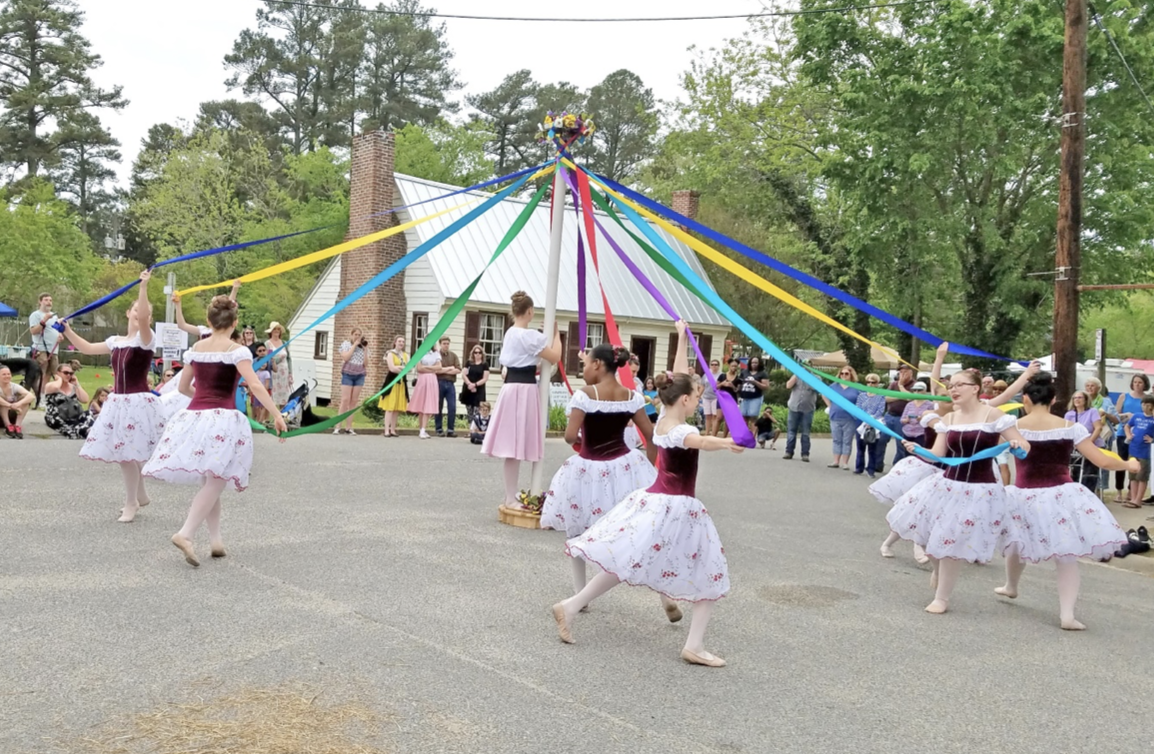In this outdoor photograph, set against a white sky, a lively maypole dance unfolds in a large paved area resembling a parking lot in front of a small white house with red brick chimneys on either side. At the center stands a girl in a white blouse and pink skirt, cinched with a black belt, guiding the performance. Surrounding her, seven young girls in burgundy velvet bodices and flowing white skirts adorned with red floral designs, all wearing white tights and ballet flats, dance gracefully. Each dancer clutches a brightly colored ribbon—red, purple, blue, yellow, or green—radiating from a flower-crowned maypole. Their hair neatly styled in buns, they weave intricate patterns as they move in different directions around the maypole. An attentive crowd of adults and children, possibly tourists, encircles the dancers, adding to the festive atmosphere, which is framed by distant greenery.